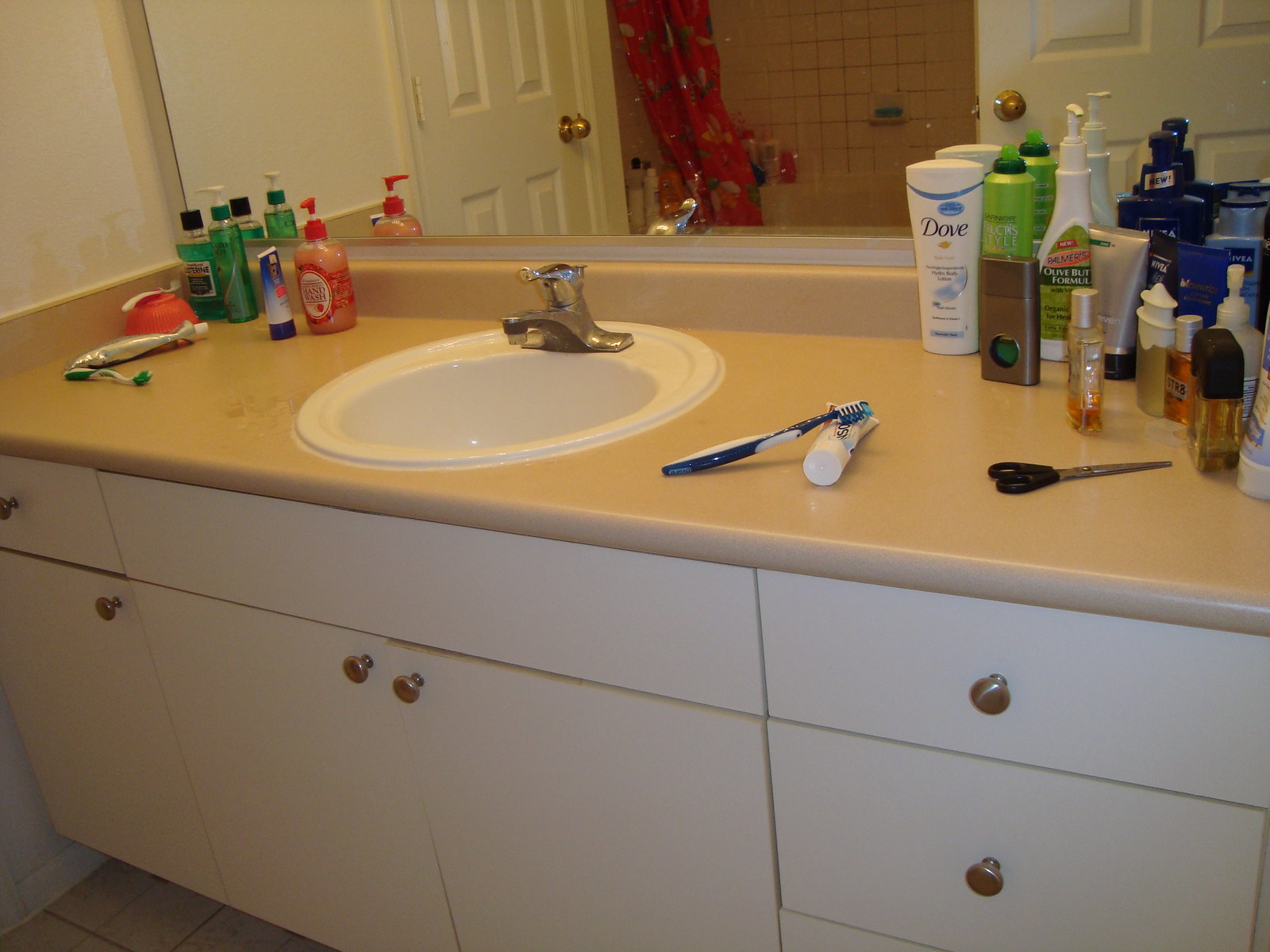This image showcases a meticulously detailed bathroom within a private residence. Dominating the top half of the image, a large mirror spans the width of the bathroom, reflecting a door, a tiled shower, and another door in sequence. Both doors feature gold-colored handles, adding a touch of elegance. The shower's walls are covered in white tiles, and a red shower curtain adorned with bug logos is also visible in the reflection, injecting a playful element into the otherwise serene space.

At the center of the image lies a circular sink with a pristine white interior, complemented by a silver faucet. The bathroom countertop is laden with various personal care items. On the left side, there's a bottle of green mouthwash, green antibacterial soap, and a green toothbrush neatly arranged. The right side of the counter holds several items, including a shampoo tube, a blue toothbrush, a pair of silver scissors with black handles, and an assortment of cologne and perfume bottles.

Beneath the countertop, the cabinetry features seven drawers with circular silver handles, providing ample storage space for bathroom essentials. The drawers' neat alignment and reflective handles echo the bathroom's clean, organized, and stylish aesthetic.